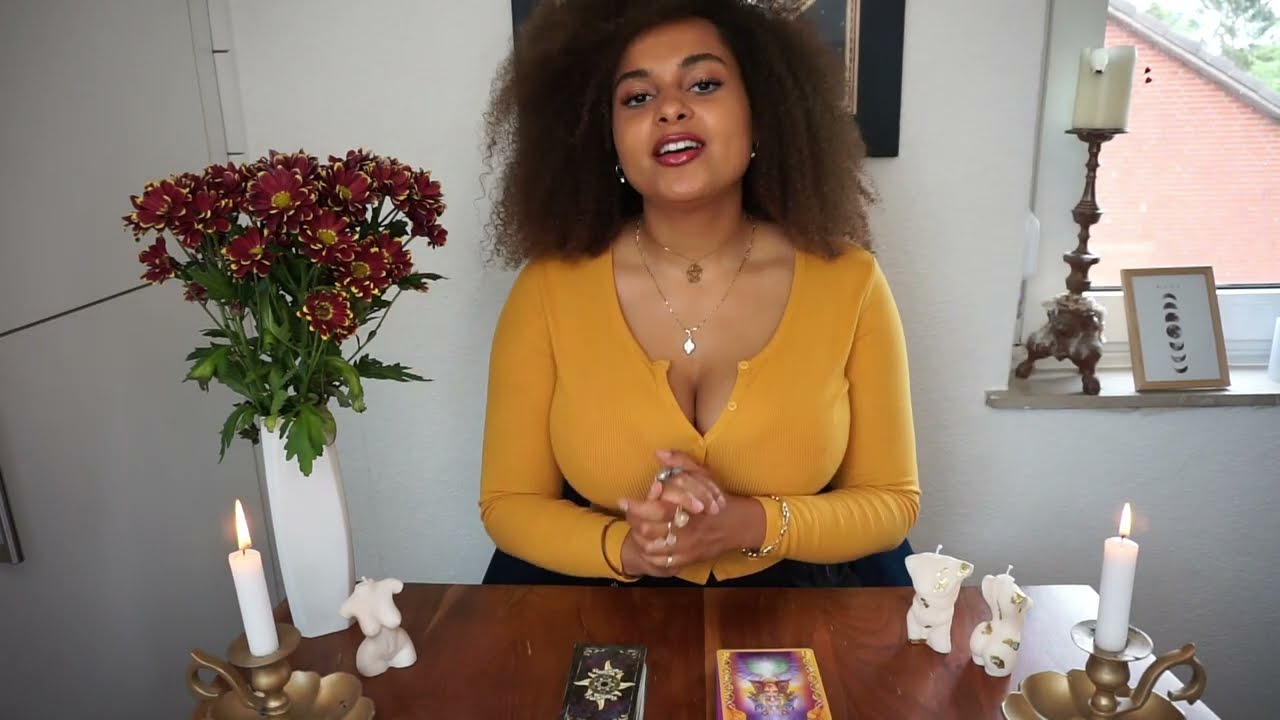In the photo, an African-American woman is sitting at a wooden table adorned with various items. She is wearing a mustard-colored, low V-neck, button-down shirt with some buttons left unfastened, revealing a generous amount of cleavage. Her outfit is complemented by a gold necklace, layered with a second gold necklace, and numerous rings on her fingers. Her hair is frizzy brown, and her lips are bright red.

The table in front of her features a white vase with red and yellow flowers, a lit candle in a candle holder on the left side, and another candle beside female torso figurines on the right. The center of the table holds a tarot deck, with some cards face up and others face down, suggesting she might be in the process of a reading. The woman's hands are clasped together, giving the impression she is about to explain something or conduct a card reading.

In the background, there is a partially visible window that looks out towards another house. On the windowsill stands a tall candle. The overall setting, along with the tarot cards and candles, suggests she might be a card reader or involved in some form of spiritual or mystical practice.